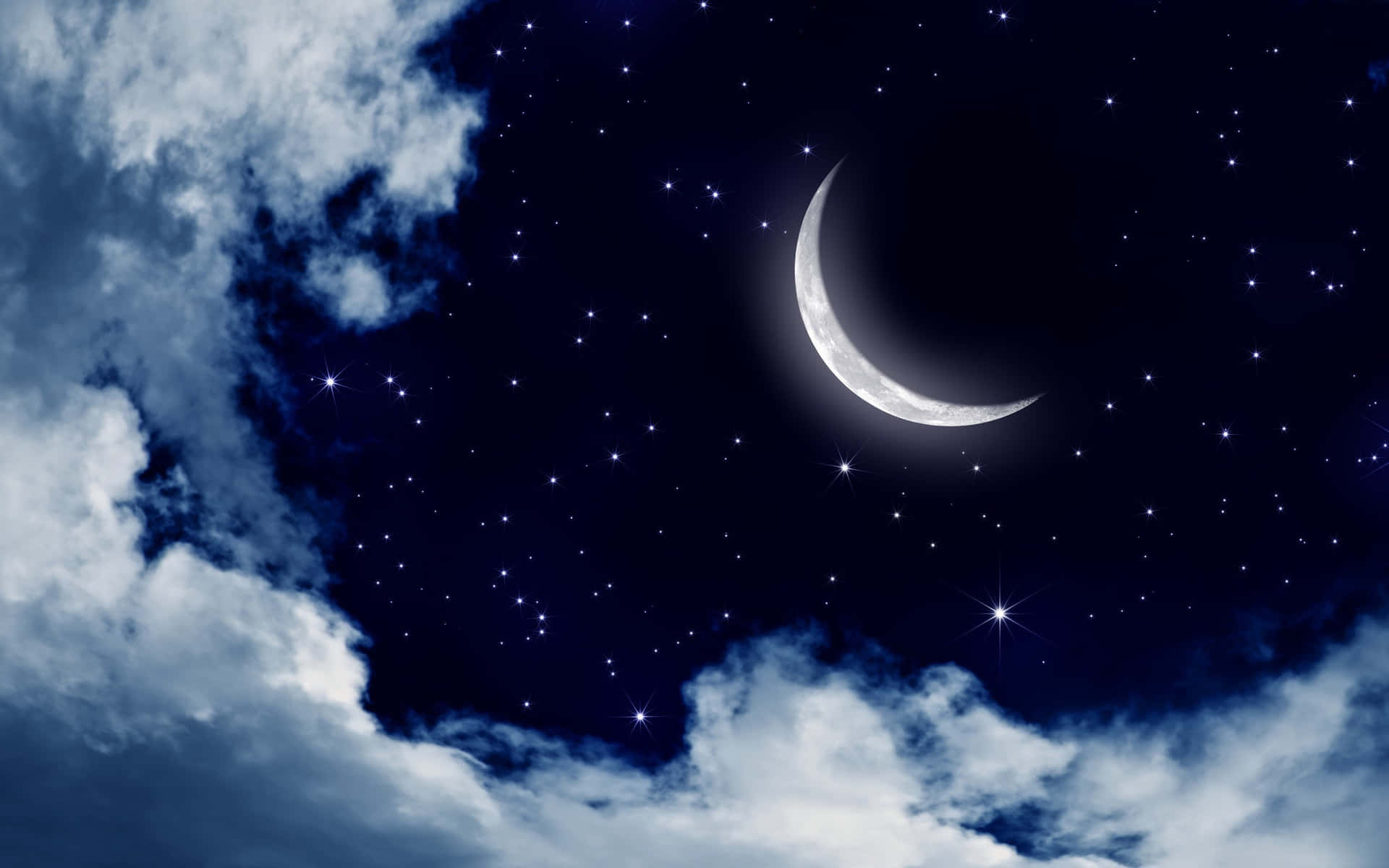This image depicts a serene night sky with a slightly navy to black background, speckled with an array of bluish and white stars, some of which exhibit a twinkling effect. In the top right center, a delicate crescent moon is visible, its slim shape slightly tilted down and to the left. A soft white glow emanates from the moon, subtly illuminating the sky around it and casting the remaining black portion of the moon against the starry backdrop, effectively obscuring the stars in that area. Framing the scene, thick cumulus clouds with a whitish-blue to bluish-white hue, interspersed with deeper blue or gray speckles, stretch from the top left, curving down to the bottom right, and partially envelope the left and bottom edges of the image. The celestial scene, whether a photograph or a realistic drawing, exudes a simple yet dramatic ambiance that evokes the quiet beauty of a starry night.